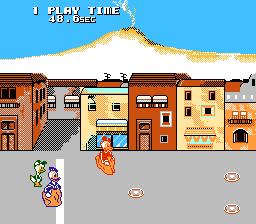This colorful illustration, likely from a simple phone or console video game, depicts a vibrant scene set against a clear blue sky. In the upper left-hand corner, white text partially reads "playtime," though the complete message is obscured. Beneath the sky, a white mountain with yellow edges adds a scenic backdrop.

Below the mountain, a row of multi-story buildings in shades of red and beige line a grey roadway that cuts across the lower part of the image. These structures feature various windows and doors, adding to the urban feel. To the left of the buildings, another roadway runs parallel, providing a pathway between the buildings and the grey road in front.

On the grey road, a vertical line marks the layout, near which two characters resembling ducks stand to the left. Another character, dressed in orange, occupies the center of the scene. Scattered on the grey ground are three small rectangles, their purpose remaining unclear, adding an element of mystery to the image.